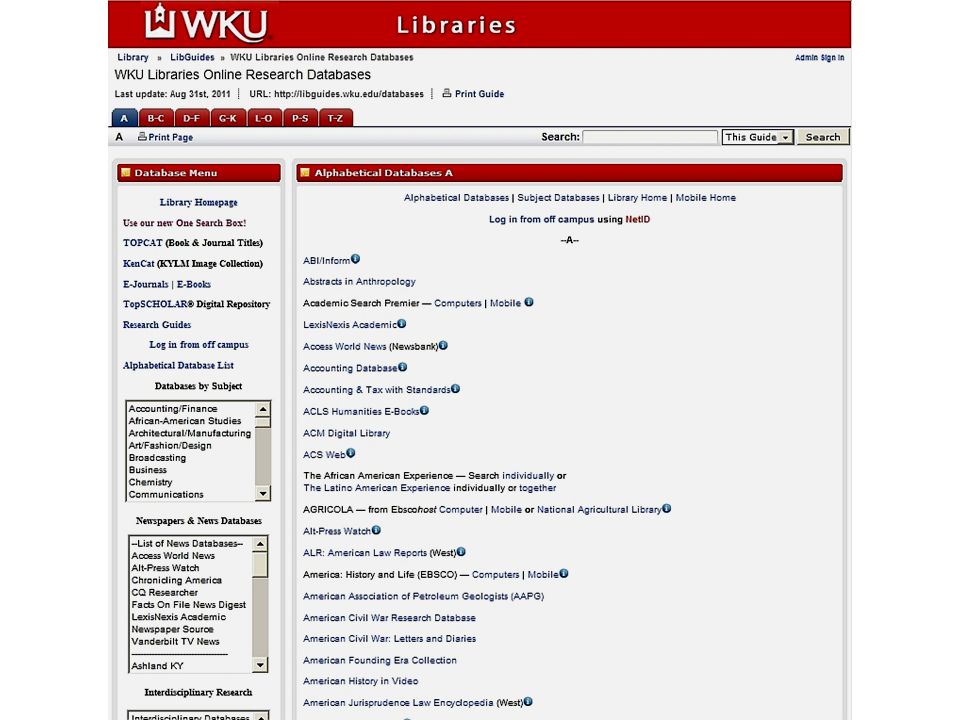The image is a screenshot from the WKU Libraries' online research database. A red banner across the top of the page prominently displays "WKU Libraries." Beneath this, there's a header that reads "WKU Libraries Online Research Databases." Below this header, there are several tabs labeled with letter ranges: A, B to C, D to F, G to K, L to O, P to S, and T to Z. The "A" tab is currently selected.

On the left-hand side of the screen, a narrower menu is visible, titled "Database Menu," with multiple options listed underneath. Occupying a larger section to the right, the main menu begins with "Alphabetical Databases A" at the top. Beneath this are additional links: "Alphabetical Databases," "Subject Databases," "Library Home," "Mobile Home," and "Login from Off-Campus using NetID."

The list of databases under the "A" tab includes the following:

- ABI/INFORM
- Abstracts in Anthropology
- Academic Search Premier
- Computers & Mobile
- LexisNexis Academic
- Access World News
- Accounting Database
- Accounting and Tax with Standards
- ACLS Humanities E-Books
- ACM Digital Library
- ACS Web Editions
- African-American Experience
- AGRICOLA
- Alternative Press Watch
- ALR (American Law Reports- US)
- America: History and Life
- American Association of Petroleum Geologists Publications
- American Civil War Research Database
- American Civil War Letters and Diaries
- American Founding Era Collection
- American History in Video
- American Jurisprudence Law Encyclopedia